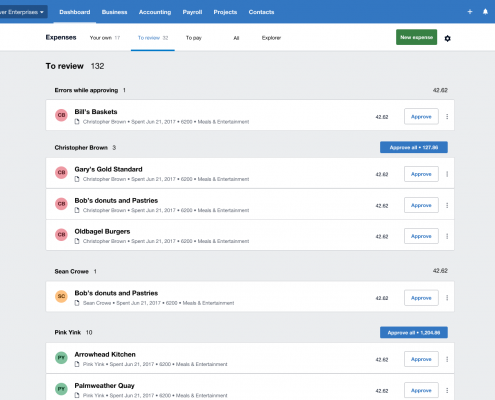This image showcases a detailed view of a business management website. At the top, there are six white categories labeled: Dashboard, Business, Accounting, Payroll, Projects, and Contacts. A notification bell icon is located in the top right corner. Below this menu, smaller categories are listed horizontally, with the third category from the left highlighted in blue. 

To the right of these categories, a green rectangle displays a message, and beneath that, the text "To Review 132" is visible. The section that follows lists several entities with a header stating "Errors While Approving." The entities listed are: Bill's Baskets, Christopher Brown, Gary's Gold Standard, Bob's Donuts and Pastries, and OK Bagel Burgers. Each entity has an associated number to the right, accompanied by a blue "Approve" button and a gray rectangular outline.

Further down, additional entities such as Sean Crow, Bob's Donuts and Pastries, Pink Yink, Arrow Kitchen, and Palm's Weather Quay are listed, each with an "Approve" button on the right. The top and bottom sections both feature an "Approve All" option. The entire layout is set against a light gray background.